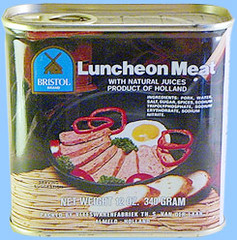The image features an off-brand SPAM can, identified as a product of Holland. The can is traditional rectangular shape with rounded edges, resembling the classical SPAM can design. It has a brass-like appearance with a convenient pop-top lid for easy opening. The brand name "Bristol" is prominently displayed on the front, set within a unique half-window shape featuring a brown windmill in the center, symbolizing the Netherlands. The background of the logo is blue, enhancing the visibility of the windmill and brand name.

The label reads "Luncheon Meat with Natural Juices - Product of Holland," indicating that the meat inside is of Dutch origin. Additional label details include the ingredients list and a picturesque illustration depicting serving suggestions. The illustration shows neatly arranged slices of luncheon meat paired with a hard-boiled egg, bell pepper, and more slices of the meat displayed on a wooden table, suggesting a versatile range of meal options. The overall presentation of the can exudes a rustic yet practical aesthetic, aligning with the traditional Dutch culinary heritage.